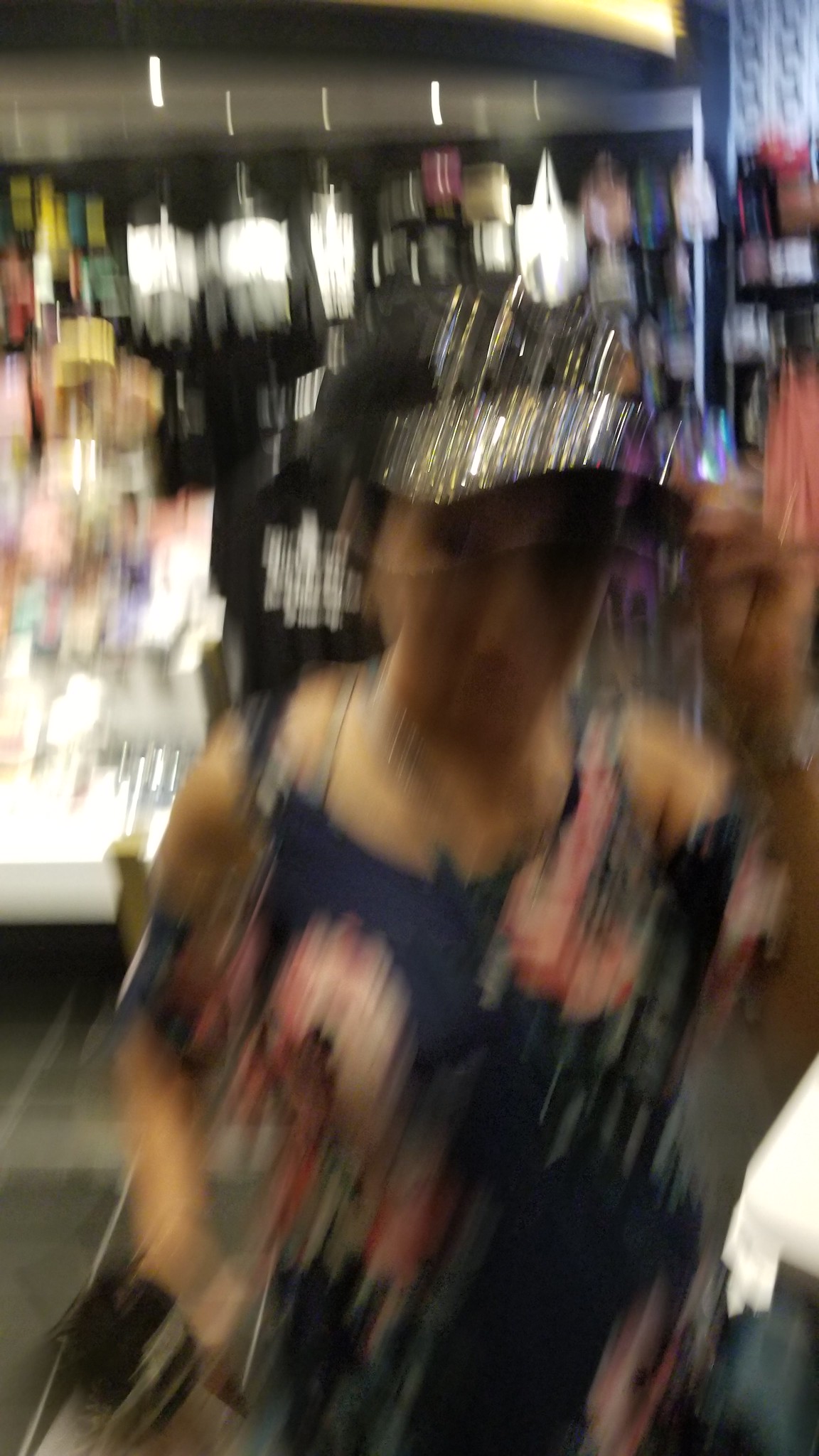The photograph is a tall, rectangular image, significantly taller than it is wide, captured indoors. The overall quality is extremely blurry, likely due to movement while the photo was taken, making specific details hard to discern. Centrally positioned in the image is a young woman, possibly Caucasian or Asian, facing the camera from the waist up. She is wearing a dark blue spaghetti strap or halter-style tank top adorned with large, light pink and potentially light orange flowers. Her outfit and appearance provide the most recognizable details despite the blurriness. The woman has a slightly tanned complexion, wears glasses, and has on a black hat with a distinctive silver brim. She appears to be holding an unidentified object in her right hand. The background suggests the photo was taken inside a store, where patterns and various fixtures, likely lighting or hanging bags, are faintly visible against a black and white backdrop, adding to the retail ambiance.